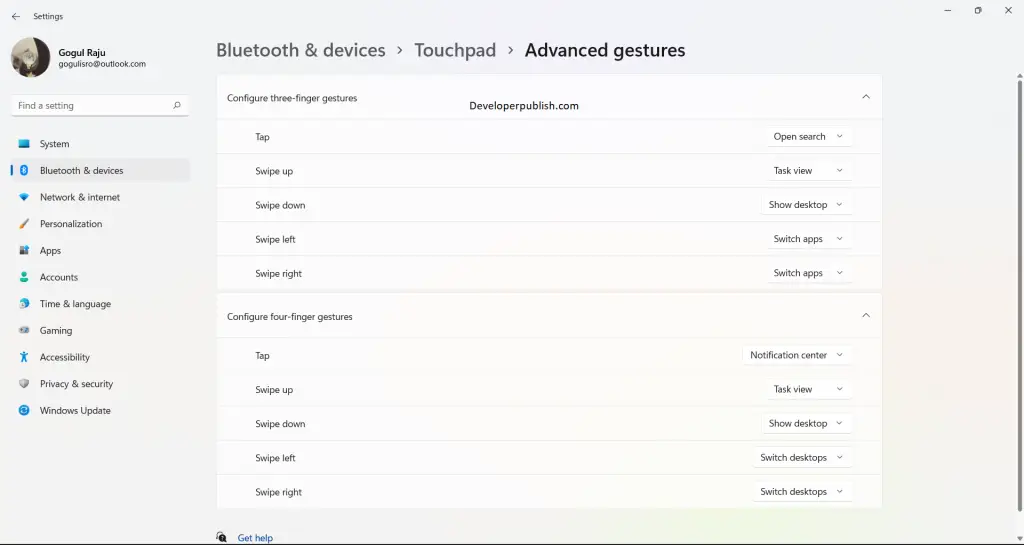This image captures a screenshot of a website detailing the configuration of advanced touchpad gestures for a computing device. At the top of the screenshot, there's a navigation trail labeled "Bluetooth and devices," followed by an arrow leading to "Touchpad," and another arrow pointing to "Advanced gestures," which is highlighted in bold. 

The main section of the page features options to configure three-finger gestures, including:
- Tap
- Swipe up
- Swipe down
- Swipe left
- Swipe right

Below this, the section lists "developerpublish.com" and continues to the configuration settings for four-finger gestures, which are:
- Tap
- Swipe up
- Swipe down
- Swipe left
- Swipe right

The detailed options for the three-finger gestures include:
- Open search
- Task view
- Show desktop
- Switch apps (listed twice)

For four-finger gestures, the options are:
- Notification center
- Task view
- Show desktop
- Switch desktops (listed twice)

On the sidebar of the page, various options are visible, including a profile picture in a circle labeled "Google, Raul," and a search box with "Find a setting." The sidebar navigation menu lists several categories:
- System
- Bluetooth and devices
- Network and internet
- Personalization
- Apps
- Accounts
- Time and language
- Gaming
- Accessibility
- Privacy
- Accuracy
- Windows update